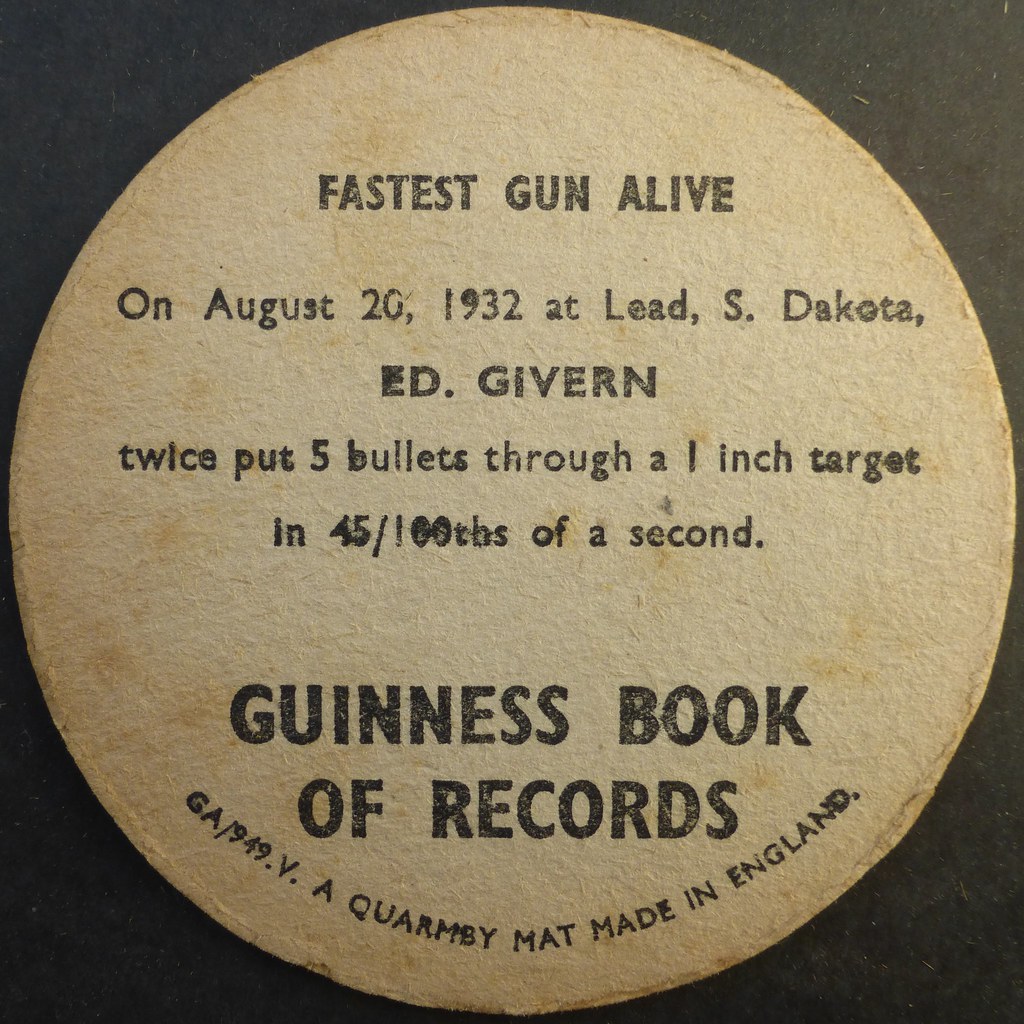This image features a square-shaped photo with a central, beige, weathered circle resembling parchment paper, set against a black or possibly dark brown background. The circle contains black writing that declares, "Fastest Gun Alive." It details an event from August 20th, 1932, in Lead, South Dakota, where Ed Givern twice shot five bullets through a one-inch target in 45 one-hundredths of a second. The text attributes this feat to the Guinness Book of World Records. At the bottom, there's a signature that reads, "GA/949.V.A. Quarmby, made in England." The circular element may suggest a seal or paper coaster.